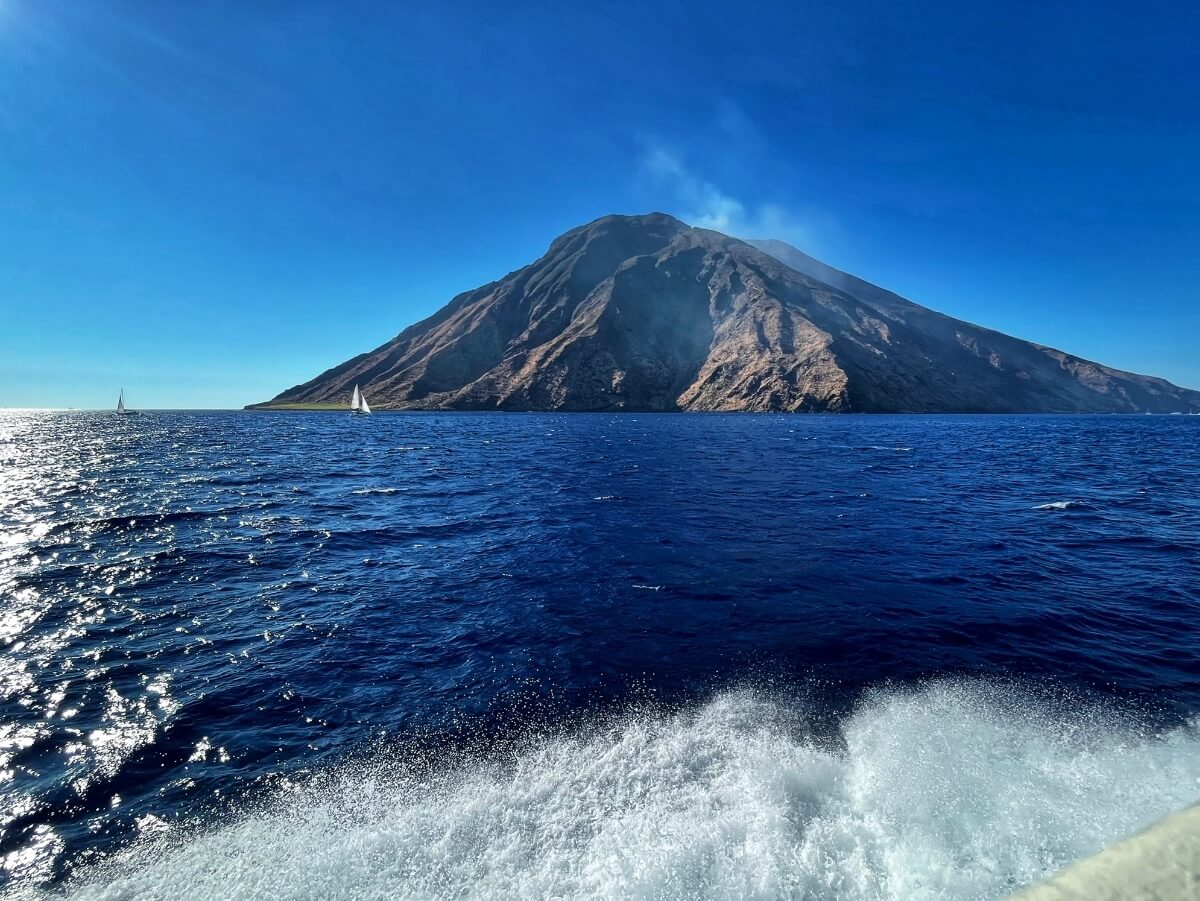This photograph, taken from a boat in the ocean, captures a stunning scene with intricate details. The deep navy blue ocean is calm but for the small ridges and white wakes caused by the boat's movement, hinting at a leisurely voyage. The dynamic foreground features splashes of seawater and a pale yellow band tracing the edge of the boat. The sunlight sparkles brightly on the water to the left.

In the background, two small sailboats can be seen on the left side of the frame, positioned towards a dramatic island. This island is dominated by a steep, dark gray and light brown mountain peak that abruptly rises from the ocean. A thin strip of green vegetation clings to the bottom left of the island, near the shore. Above the mountain, wispy white clouds drift in a serene deep blue sky, adding to the sense of tranquility on this beautiful, sunlit day.